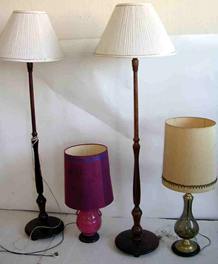This photograph showcases four distinct lamps arranged in a store display against a bifurcated background with a beige upper wall and a white lower section. The surface beneath the lamps is also white. The two tall floor lamps, positioned on the left and second from the right, feature slender metal bases with round bottoms, finished in dark brown or black. Their white lampshades, which narrow slightly towards the top, appear proportionally short for their tall bases. In the center is a small, visually striking table lamp with a pinkish-purple, globe-like glass base and a dark purple, tubular shade on a round black base. The fourth lamp, situated on the far right, is another table lamp, distinguished by its vase-shaped green glass base atop a brass bottom. This lamp is adorned with a burlap shade that has a light band trimming around its bottom edge. The composition of lamps, differing in height, color, and design, creates an intriguing contrast against the minimalist background.